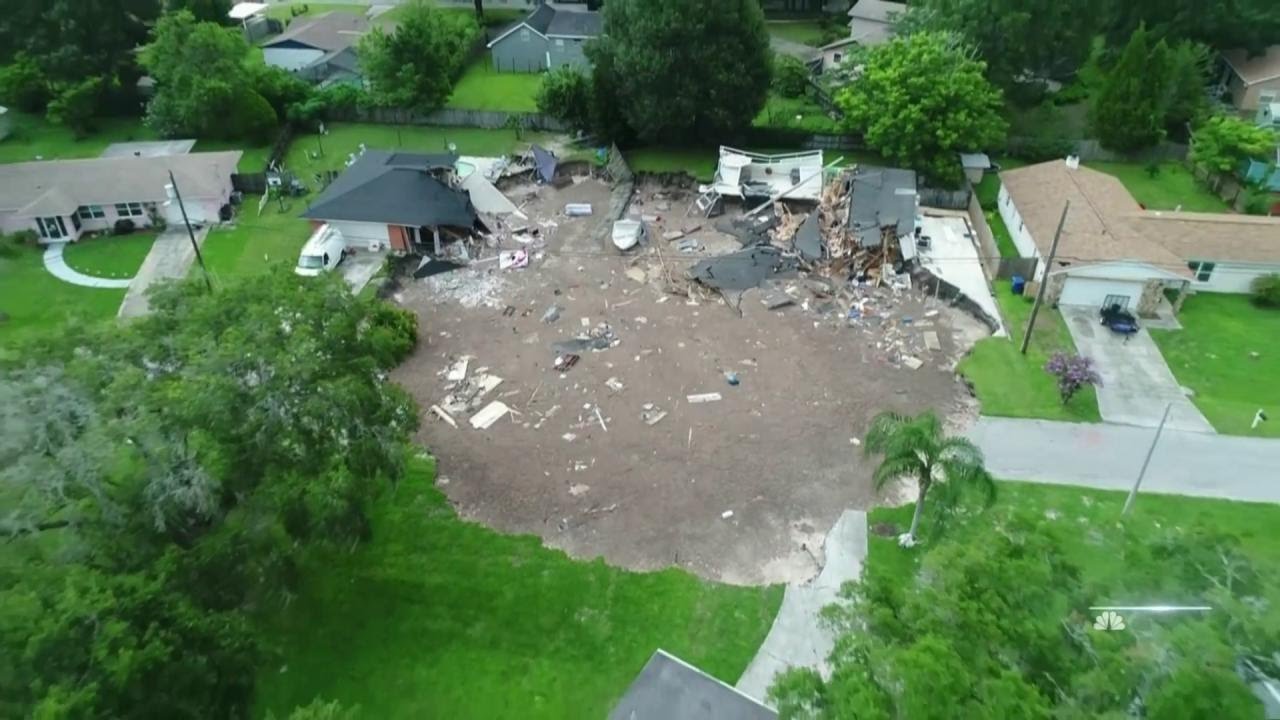This aerial daytime photograph captures a suburban neighborhood, where a devastating scene draws immediate attention. Centered in the image, an entire house has been obliterated, likely due to a tornado. The circular plot where the house once stood is now a barren patch of earth, scattered with debris ranging from structural materials to personal belongings. Surrounding this destruction, the lawns remain green, indicative of the tornado's selective fury that spared the neighboring homes. To the left of the demolished site, remnants of what appears to be a still-standing garage can be observed. Various houses in the vicinity feature distinct architectural styles, including one-story white-walled homes with Spanish-style pink tile roofs, and manicured lawns. The photograph shows a mix of trees, including a palm tree on the lower right and regular green-leaved trees on the left, creating a stark contrast with the destruction in the center. A crisscross pattern on the grass surrounding the affected area further highlights the normalcy disrupted by the disaster. In the bottom corners of the image, roads and driveways are visible, accentuating the suburban setting of what appears to be a semi-rural area, now marked by the tragic and violent impact of the tornado.